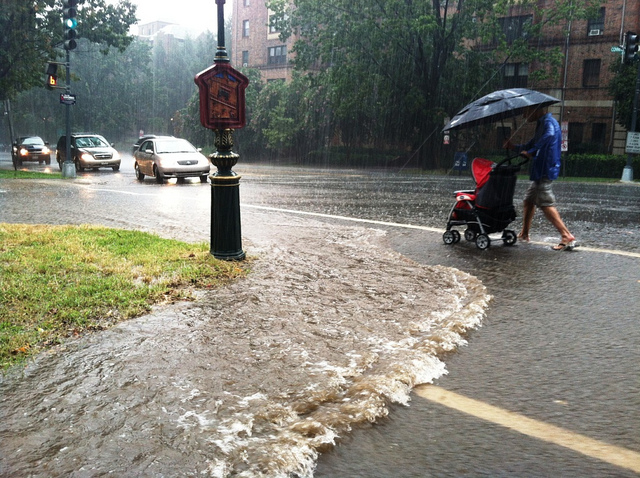The image is a color photograph capturing a dramatic street scene during a heavy storm. The central focus is a person walking along the edge of a flooded black asphalt road, pushing a six-wheeled black baby stroller with a red canopy. The person is partially visible, dressed in a blue jacket, beige shorts, and blue flip-flops, and holding a large black umbrella that shields both them and the stroller from the downpour. The road is marked with white solid lines on the edges and a yellow stopping area line, with brown, muddy water and white foam accumulating on the street's flooded shoulder. 

Adjacent to the road, on the left side, is a heavily flooded area, where water is overflowing next to a small green side mound and green grass. In the background, the photograph reveals a multi-storied brick apartment building partially obscured by large green trees. Trees hide some windows, adding to the stormy ambiance. Cars with their headlights on are visible on the left side of the image, driving cautiously through the stormy weather. A street marker with a house-shaped placard extends from the center to the top of the image. Above, the sky is a uniform white, showing the severity of the rainstorm that dominates the scene. The photographic style is representational realism, capturing the raw, unpredictable nature of the cityscape under such extreme weather conditions.